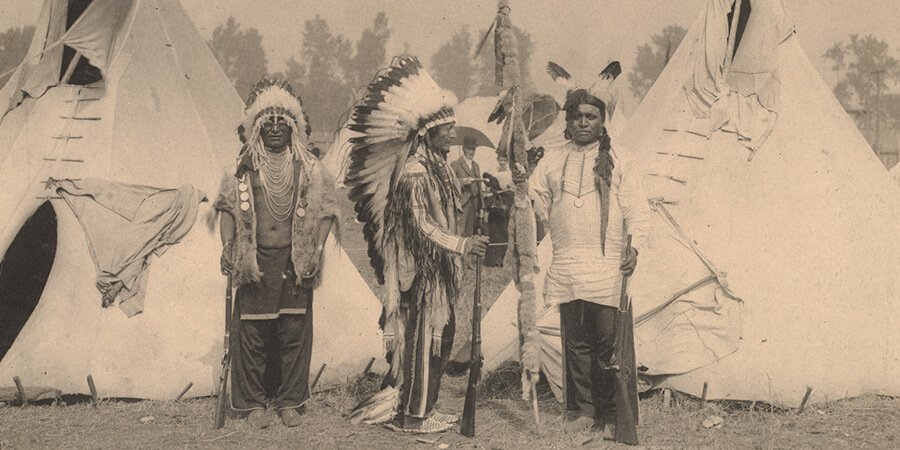This black and white photograph, possibly from the early 1900s, depicts three Native American men standing in traditional attire. The image is horizontally oriented like an old photograph, with a slightly pinkish background tint. 

### The Men:

1. **Leftmost Man:**
   - **Attire:** He wears a detailed headdress with white and red feathers.
   - **Clothing:** A vest adorned with numerous necklaces, with no shirt underneath, and dark pants.
   - **Weapon:** Holds a rifle in his right hand, with the rifle butt resting on the ground.

2. **Middle Man:**
   - **Attire:** Donned in a brown leather top and dark pants that possibly have stripes.
   - **Headdress:** A long headdress with white feathers and dark tips extending well below his waist.
   - **Weapon:** Carries a rifle in his right hand, barrel up and butt on the ground.

3. **Rightmost Man:**
   - **Attire:** Sports long hair over his left shoulder, a white shirt or apron, and dark pants.
   - **Garment:** Holds a long stick adorned with furs or small animals in his right hand.
   - **Weapon:** Similarly, holds a rifle in his left hand, with the rifle butt resting on the ground.
 
### Background:

- **Teepees:** There are two teepees, one on each side of the image, with openings visible.
- **Figure in the Background:** A man wearing a suit and a top hat stands between the teepees.
- **Scenery:** A row of trees is visible at the top background of the image, above the grass and dirt ground.

The detailed attire, the traditional weapons, and the presence of teepees underscore its depiction of Native American culture, making this a fascinating historical photograph.